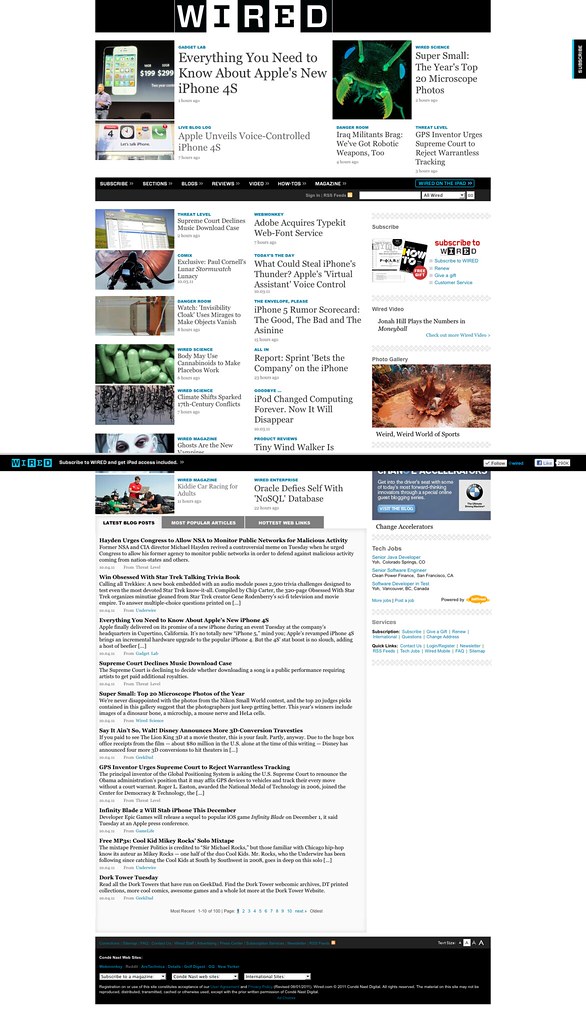In this image, you see the homepage of the Wired website featuring various news headlines. Prominently displayed is a headline about Apple's new iPhone 4S, emphasizing its voice-controlled capabilities, which include the much-talked-about virtual assistant. Other major headlines include a story titled "Everything You Need to Know About Apple's New iPhone 4S" and another on "Adobe Acquires Typekit Web Font Service." There's a headline discussing the Supreme Court's decision regarding music download paces, as well as an article on Iraq militants boasting about robotic weapons. Additional stories cover diverse topics such as the rejection of warrantless tracking by the GPS inventor, mind-bogglingly small photographs in the US Top 20 Microscope Photos, and a feature on an invisibility cloak that uses mirages to make objects disappear. The lineup continues with intriguing topics like the body's use of cannabinoids to make placebos work, a climate shift that sparked 17th-century conflicts, and cultural pieces, including "Ghosts Are the New Vampires" and "Tiny Wind Walker."